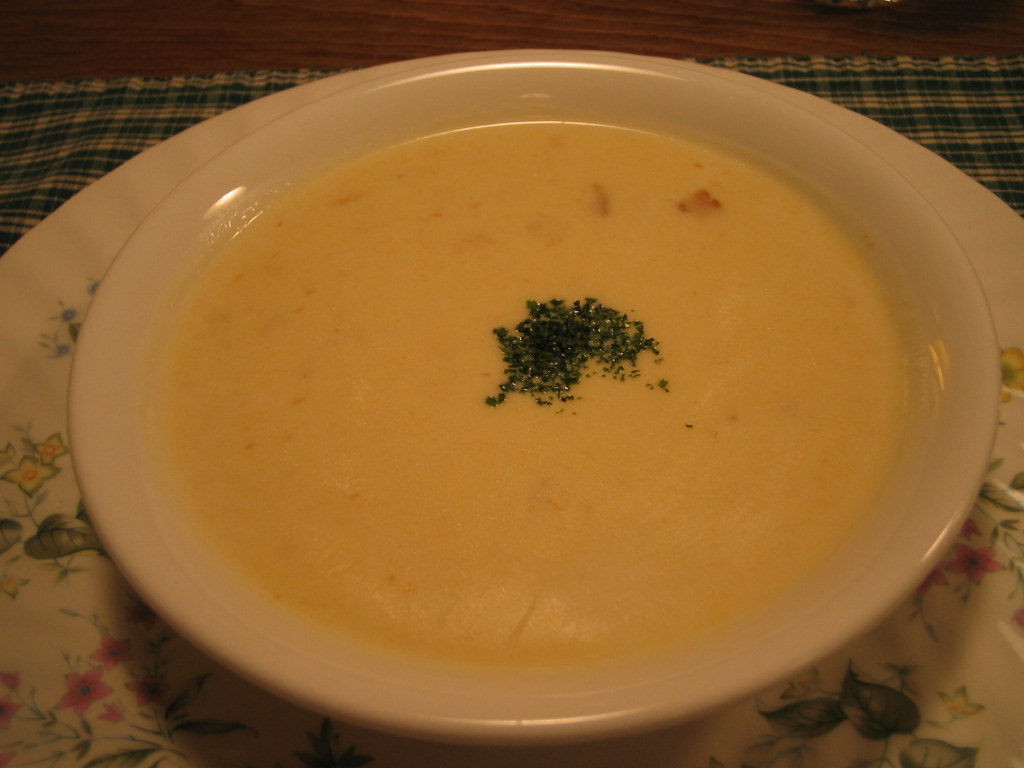The photograph showcases a bowl of yellowish-tan soup with various pink squares floating in it, garnished with chopped green herbs, possibly parsley or chives, sprinkled in the center. The soup is served in a white porcelain bowl with rounded edges, which is placed on a larger porcelain plate. The plate features a floral design with pink, white, and blue five-star shaped flowers, and possibly some green leaves, and it has scalloped edges. This ensemble is set on a blue and white plaid placemat, which rests on a light brown wooden table, adding a rustic touch to the presentation. The colors in the image include shades of yellow, white, green, pink, blue, and brown, creating a harmonious and inviting scene.